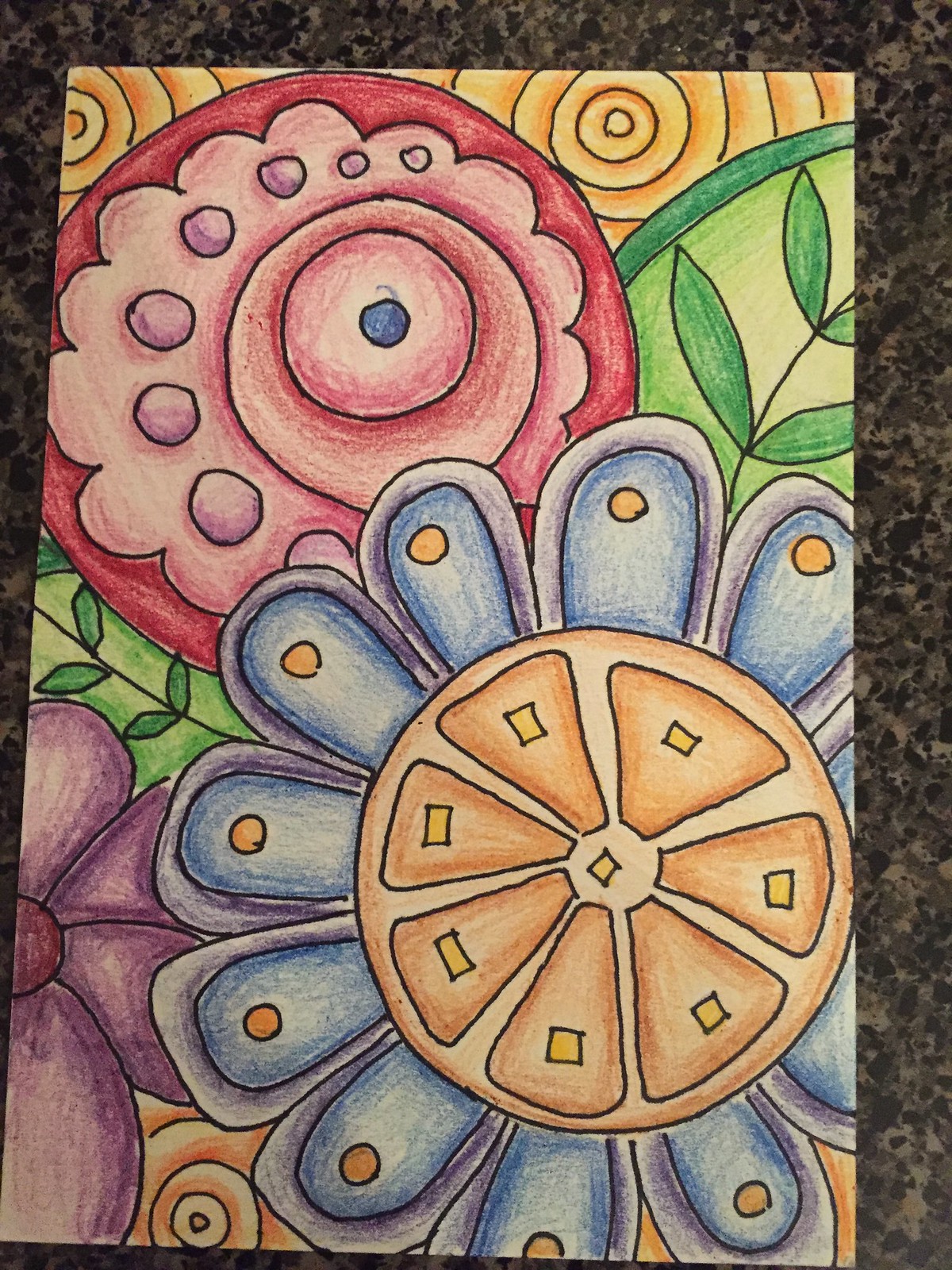A vibrant, colored pencil drawing is prominently displayed on a countertop, as indicated by the visible texture in the background. The photograph captures the artwork from a top-down perspective, allowing for an in-depth view of the intricate details. The drawing features several round shapes, each distinct in design and color. In the bottom right corner, there is a detailed representation resembling a grapefruit with striking blue petals. On the top left, a large circle seemingly depicts a rose adorned with a central blue dot, adding a unique touch to the composition. Additionally, a portion of an actual flower is partially visible on the bottom left side of the image, introducing an element of realism to the artistic display.